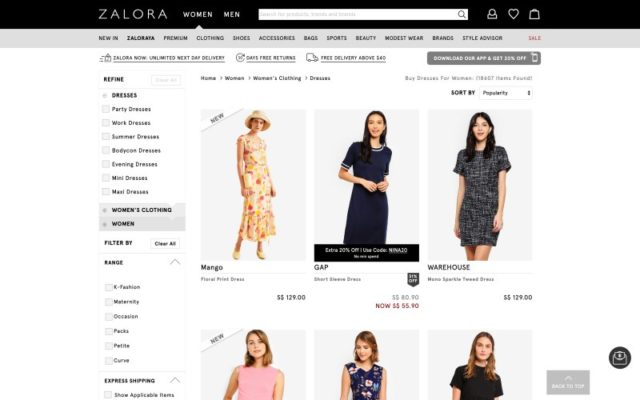This screenshot showcases a meticulously designed Zalora website interface. At the very top, a sleek black banner features crisp white text. On the upper left, the Zalora logo is prominently displayed. Adjacent to it, smaller white text options read "Women," "Men," and include a white search bar for easy navigation. Further to the right, icons for a user profile, favorites (heart icon), and a shopping bag enhance user interactivity.

Below this, a gray secondary banner spans the width of the screen, listing categories in black text: "New In," "Premium," "Clothing," "Shoes," "Accessories," "Bags," "Sports," "Beauty," "Modest Wear," "Brands," and "Style Advisor." To the far right, the eye-catching word "Sale" is highlighted in red.

In the main content area, six vibrant images feature stylish young women showcasing the latest fashion trends. Starting from the top left, the first image displays a woman in a calf-length yellow dress with short sleeves and a hat, captioned "Mango." To her right, a woman dons a dark dress, labeled "Gap." The next image features a young woman with black hair wearing a short-sleeve, short dress, branded "Warehouse."

Each element of the website is carefully structured to provide an intuitive shopping experience, making it easy for users to explore Zalora’s diverse fashion offerings.